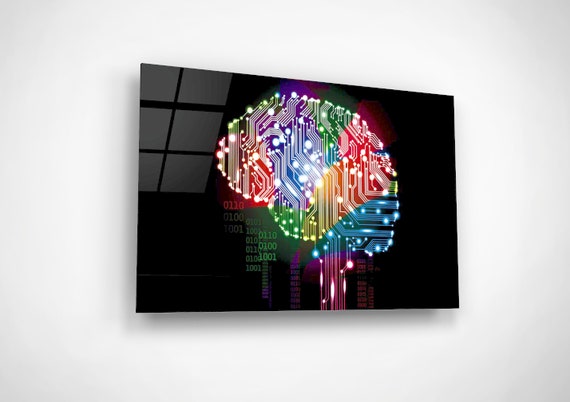This indoor color photograph captures a mounted image on a pristine white wall, possibly at a gallery. The artwork itself presents a shiny, glossy black surface that resembles either a monitor or glass. Central to the image is a detailed, intricate silhouette of a human brain. The brain is artistically represented with multicolored circuit board designs, integrating shades of red, green, blue, and yellow. These colors suggest the complex neural connectors and electric signals synonymous with the human mind. A noticeable purple stem extends downward, fading off to the right. The brain's structure is enhanced by binary code trailing off from the left, further emphasizing a blend between biological and technological elements. Additionally, reflections of a six-panel window, particularly the three left panels slightly beyond the edge of the artwork, can be observed, adding to the reflective, shiny nature of the piece.